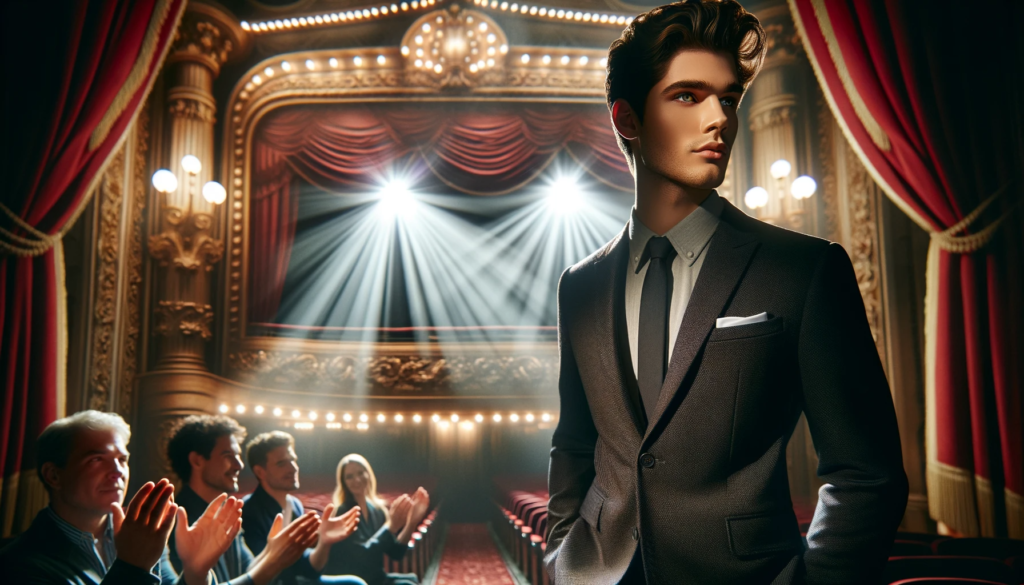This image, likely a digital artwork, depicts the interior of an ornate theater. The theater features elegant architecture with an array of red carpets and drapes accented by gold trim and small white lights. A prominent stage or screen is set at the back, illuminated by bright spotlights. In the foreground, standing to the right, is a young, handsome man with a perfectly coiffed hairstyle, wearing a brown suit paired with a white shirt and brown tie. His expression is blank, and he gazes off to the side with his hands in his pockets. Seated to the left are four individuals – three men with short hair and one woman with long hair – all clapping. The older man sits furthest left. The image captures a moment of appreciation in a richly decorated, intimate theater setting.